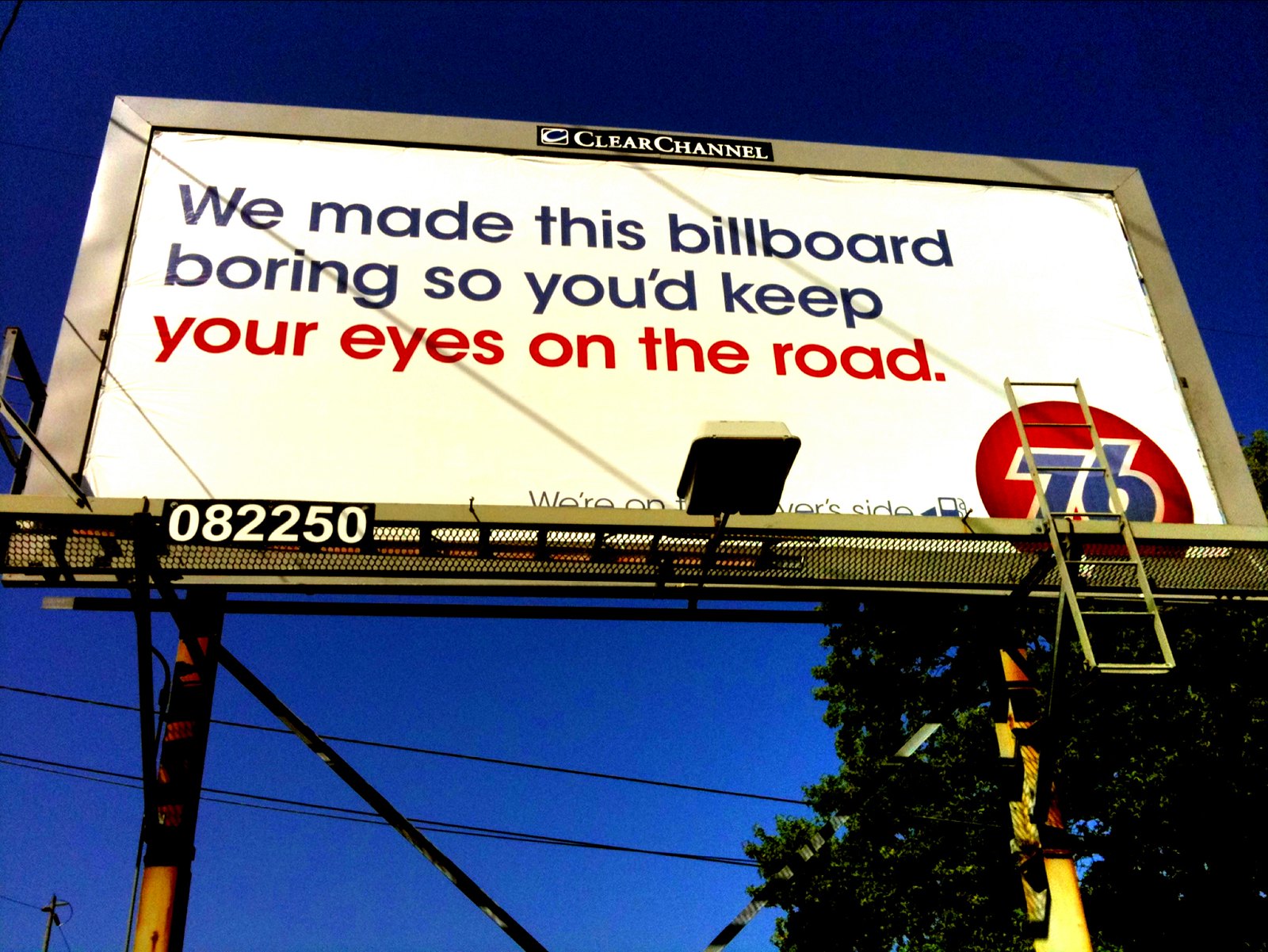This photograph captures a towering billboard from a low-angle perspective, emphasizing its substantial size and structure. The billboard features a sleek silver metal frame, accentuating its modern design. At the very top, a navy blue banner displays the text "Clear Channel" in crisp white lettering, denoting the advertising company. The main billboard area boasts a clean white background with prominent, eye-catching text. The message reads, "We made this billboard boring so you'd keep," in navy blue font. Following this phrase, "Your eyes on the road" is highlighted in bold red font, reinforcing the importance of undistracted driving. 

Situated in the bottom right corner of the billboard, a red circle encloses the recognizable Phillips 66 logo, adding a splash of brand identity. Below the billboard, a green ladder is securely attached to the lower portion of the structure, suggesting maintenance or access. The billboard is supported by two vibrant yellow posts, which stand out against the vivid blue sky. Additionally, black electrical wires traverse the background, and a green tree peeks into the frame, adding a touch of nature to the urban scene.